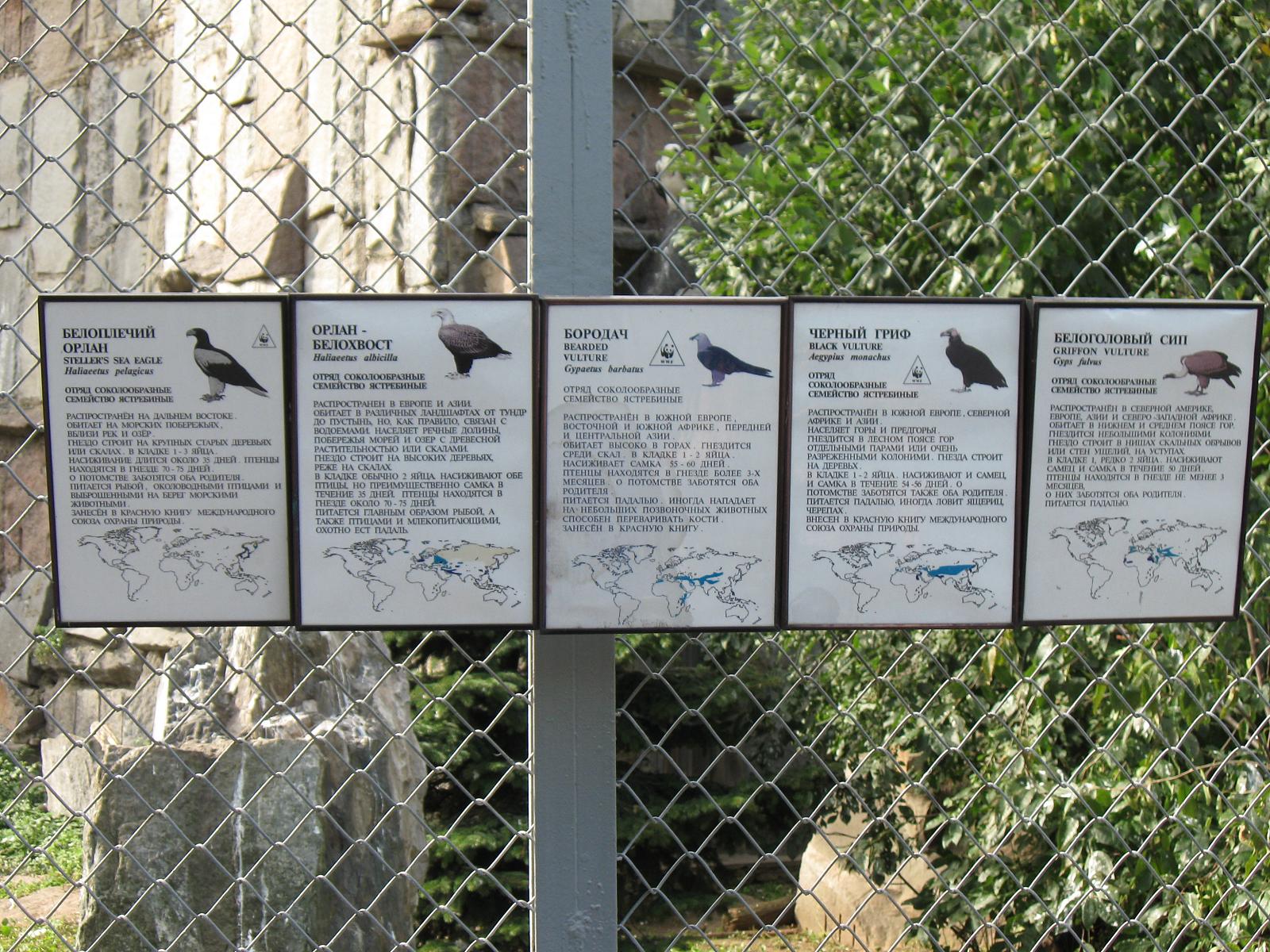The photograph depicts a typical chain link fence with two gray-painted metal pillars serving as dividers. Affixed to the fence are five framed sheets of paper, each dedicated to a different bird. On the upper right corner of each sheet is an image of the bird, with the bird's name listed on the left and additional information provided below, likely in the Russian language. At the bottom of each sheet, a world map highlights, in light blue, regions where these birds can be found. Behind the fence, an outdoor exhibit resembling a bird sanctuary is visible, featuring a naturalistic setting with trees, rocks, and grass, though no birds can be specifically seen. This setup suggests a contained yet open environment possibly designed to mimic the birds' natural habitat.